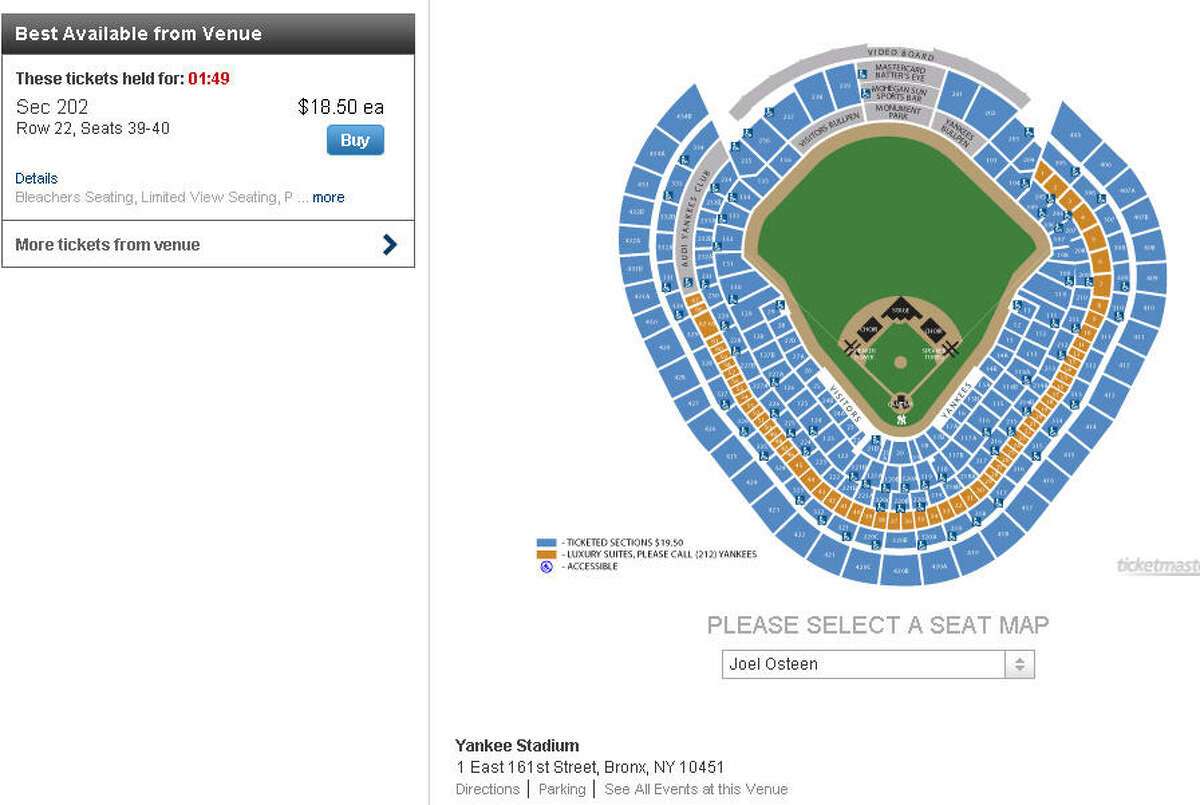In this image, we have a comprehensive view of a ticket purchasing screen for an event at Yankee Stadium. On the left side, there is a black background with white text stating "Best available from venue." Below, within a black box with white font, a timer reading "These tickets held for 01:49 minutes" is displayed. Directly beneath that information, it lists "Section 202, Row 22, Seats 39 to 40," indicating the specific seating details.

To the right of the seating information, the ticket price is shown as "$1850 each" in a clear, prominent manner. A blue button with white text labeled "Buy" appears next to the pricing for immediate purchase action.

Underneath this price section on the left, the word "Details" is in blue font, followed by gray text highlighting features like "Bleacher seating, Limited view seating," and an abbreviated note ending with "P...". Next to these details, there is a "More" option in blue font.

Further down, a horizontal black line separates the previous section from another detail that reads "More tickets from venue" in black. Next to this text, a double black arrow points to additional options.

A vertical gray line segments this portion from a visual representation of the stadium's seating plan. The seating chart includes a green baseball field with brown baselines creating a diamond shape, surrounded by blue and orange seating areas. There is also a nearly complete gray circle outlining the field. Additional details include a second lower section of blue and orange seats, enclosing a small blue circle.

In the bottom section, small gray font reads "Ticketmaster." Directly beneath it, in gray font, the instructions "Please select the seat map" can be seen. Finally, "Joel Osteen" appears with an adjacent gray up and down arrow. The bottom left of the image provides the location as "Yankee Stadium, 1 East 161 Street, Boston, New York, 10451," followed by "Directions/Parking/See all events at this venue" in gray text.